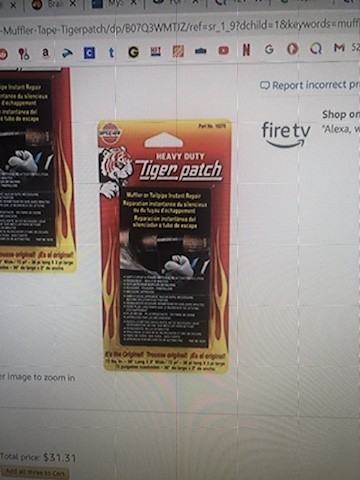The image is a detailed photograph of a computer screen displaying a product page on Amazon.com, accessed via Google Chrome. The URL at the top contains the words "muffler tape tiger patch" along with a string of letters and numbers. The page prominently features a rectangular product image labeled "Heavy-Duty Tiger Patch" in white text on an orange background that resembles flames. The packaging is designed to hang on a rack, complete with a punch-out hole. A small white tiger illustration is visible on the packaging. Additional text details are too small to decipher. To the right of the screen, "Fire TV" is mentioned, while "Shop Online" and "Alexa" are also visible. The bottom left corner shows a total price of $31.31 and includes a button to add the item to the cart. There are some partially visible, cut-off texts near the price, and a zoom function for viewing the image is suggested. At the top right corner, there's an option to report incorrect product information.